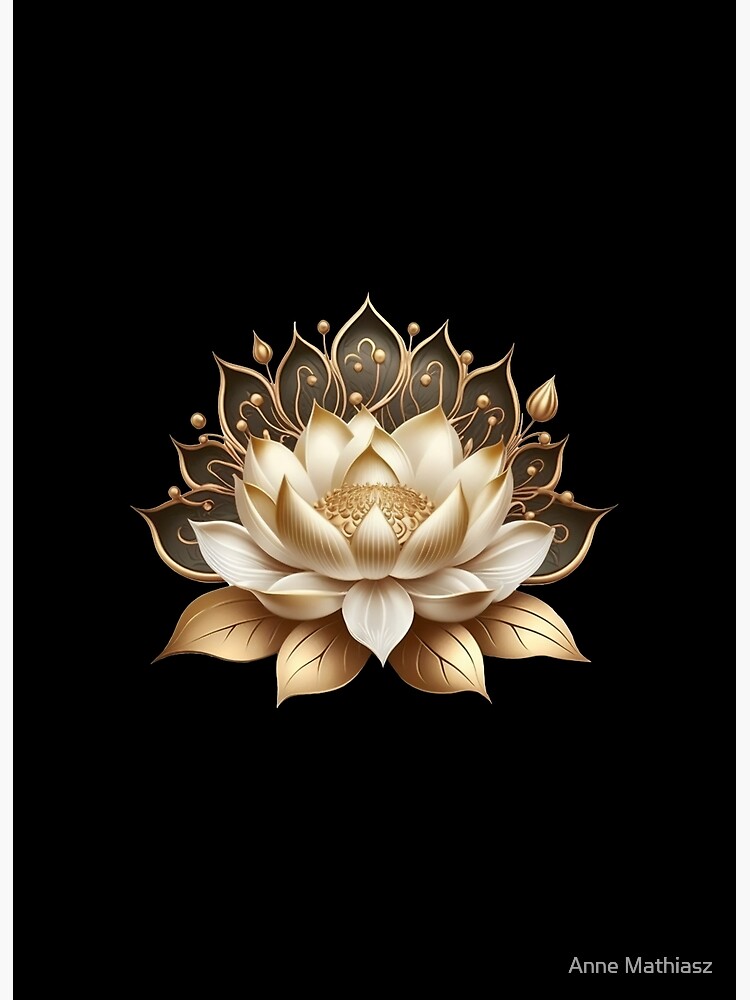This is a detailed, computer-generated image of an exquisitely designed flower, most likely a lotus. The predominant colors are white and gold, with the flower's petals primarily white tipped with tan or gold hues. The center of the flower is round, featuring intricate details. Surrounding the flower are four gold leaves with visible veins, adding to the decorative elegance. Behind the flower, there is a decorative backdrop that appears to include gold tulip-like shapes and an almost crown-like outline. The entire image rests on a black background that also has gold trimming, enhancing the flower's prominence. In the bottom corner, the artist's name, Ann Mathias, is elegantly inscribed, attributing the artwork to her.